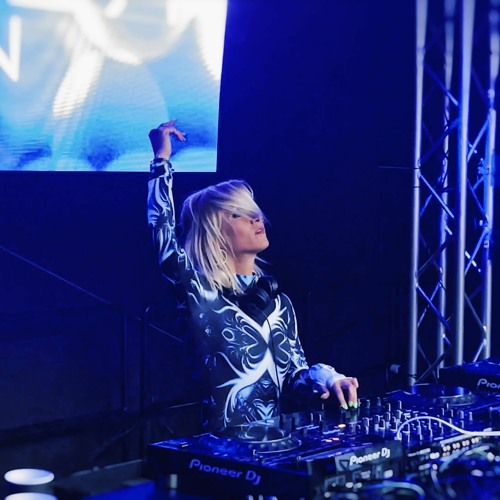The photograph captures a female DJ with dirty blonde hair, partially covering her face, performing a live set. She is dressed in a predominantly black hoodie featuring white patterns. Her fingernails are painted light green. The woman stands behind a DJ board branded Pioneer DJ, which occupies a significant portion of the right side of the image. Her right hand manipulates the dials on the board while her left hand is raised in the air, giving the impression she is deeply immersed in her performance. A pair of black headphones rest around her neck, her eyes closed as if she is in a trance. 

The environment is bathed in cyan lighting, giving both the background and foreground a distinctive tint. Behind her, a large LCD screen dominates the scene, casting a bright glow in the dark setting. To the DJ's left are two glasses, with one partially cut off in the frame. On the right side, scaffolding with silver bars extends to the ceiling, likely supporting lights or other equipment. This detailed setting suggests she is in the midst of an energetic party or nightclub event.